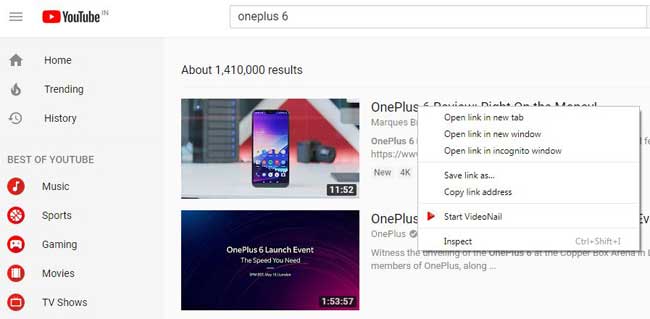This screenshot captures a detailed view of a YouTube web page. At the upper left-hand corner, the interface includes the YouTube logo and a menu icon represented by three horizontal grey lines. The partially visible address bar contains the text "1 plus 6."

Beneath the YouTube logo, a vertical drop-down menu displays options such as Home, Trending, and History. Further down, under the "Best of YouTube" section, there are red icons labeled Music, Sports, Gaming, Movies, and TV Shows.

In the main content area, two search results are displayed. The first result showcases an iPhone against a grey, white, and red background, with a duration of 11 minutes and 52 seconds. Below this, the second result is titled "1 plus 6 Launch Event," set against a purple and blue background, and runs for 1 hour, 53 minutes, and 57 seconds. Descriptive text accompanies each video thumbnail.

Overlaying these search results is a pop-up context menu with the following options listed from top to bottom: Open Link in New Tab, Open Link in New Window, Open Link in Incognito Window, Save Link As, Copy Link Address, Start Video Nail, and Inspect. Notably, a red right-facing arrow precedes the "Start Video Nail" option.

The rest of the background is white, and the image itself has no border, presenting a cleaner, minimalist appearance.